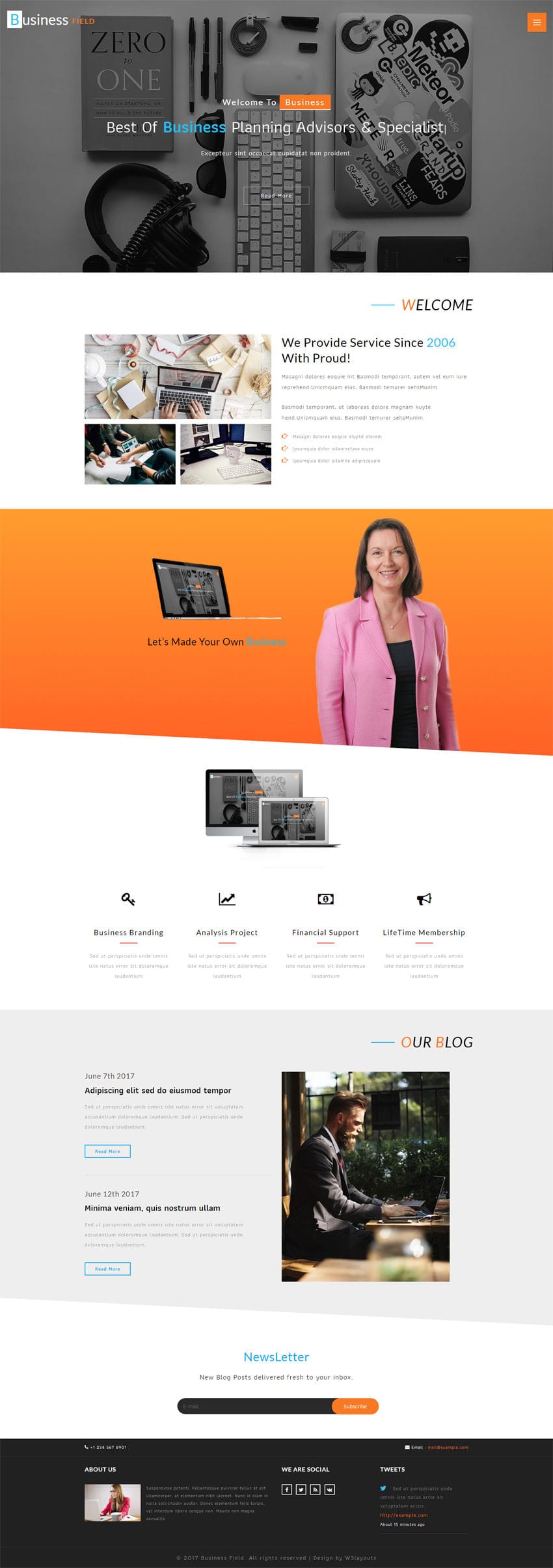This is a detailed description of a business-oriented website template available for purchase. The template features a full-scroll layout, allowing you to view the entire website design from top to bottom within a single frame. This comprehensive view enables potential buyers to understand the complete structure and aesthetic of the template.

At the top, there is a hero image, currently grayed out, intended to be the focal point upon entering the site. This image is overlaid with a grid layout displaying various items such as a book, headphones, sunglasses, and a keyboard, organized neatly within the grid. At the center of this hero section, there is a welcoming message that appears to say "Welcome to [something related to business]," accompanied by an orange call-to-action button labeled "Best of Business Planning Advisor and Specialist."

Below the hero section, the template showcases three images depicting various office activities, emphasizing the practical applications of their business services. Accompanying these images is a textual overlay that reads, "We provide service since 2006 with pride" (technically stating "with proud," which seems to be a grammatical error).

Further down, there is an orange section featuring a woman wearing a pink blazer. She has medium-length hair and is working on a laptop. The text in this section contains another grammatical error, reading "Let's made your own business" instead of "Let's make your own business."

Beneath this, the viewer sees an Apple desktop monitor with an Apple laptop positioned in front, displaying the website in different formats. This part of the template is accompanied by four small icons representing various branding options, though the specific text accompanying these icons is not legible.

Continuing down the page, the template includes a section featuring a man with a beard using a laptop, alongside two blog article placeholders with "Read More" links. At the very bottom of the template, there is a newsletter subscription section and a footer containing space for address and contact details.

Overall, this template is designed to provide a professional and organized layout for businesses looking to establish a robust online presence, despite a few minor grammatical issues that could be easily corrected.